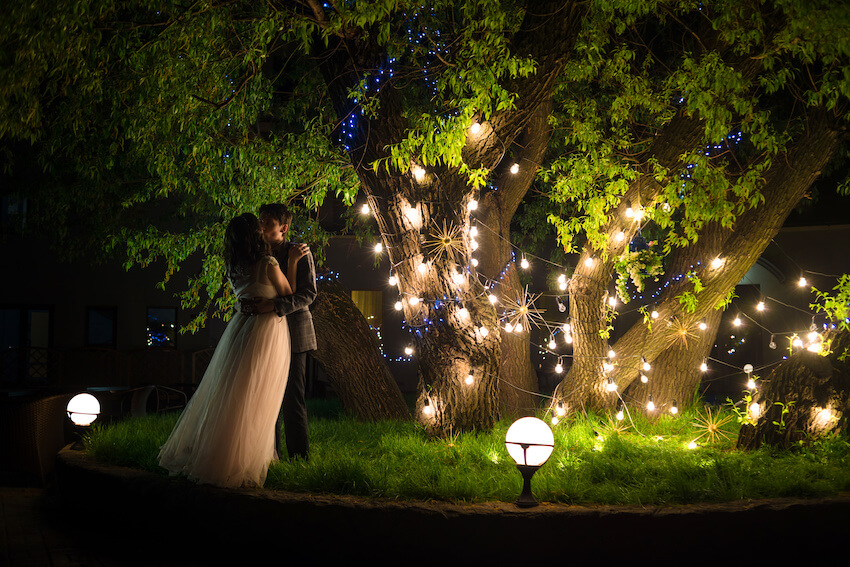Amidst a romantic nighttime setting, a young couple shares a tender kiss. The woman, with her long curly brown hair cascading over her shoulders, is dressed in an elegant white gown that could easily be mistaken for a wedding dress. Her partner, a man with short brown hair, is smartly dressed in a gray suit. They stand intimately close, holding each other—his arms around her waist and her arm resting on his shoulder.

The couple is situated on a raised tree bed adorned with five robust trees, each decorated with an enchanting mix of white and blue string lights. The lights illuminate the green leaves, casting a soft, magical glow around them. The scene is further set against the backdrop of a large building, adding to the urban charm of the setting. A cement sidewalk encircles the tree bed, marking the boundary of this picturesque spot. The atmosphere suggests a moment of celebration or deep affection, perhaps even an engagement, making it a truly captivating and unforgettable scene.